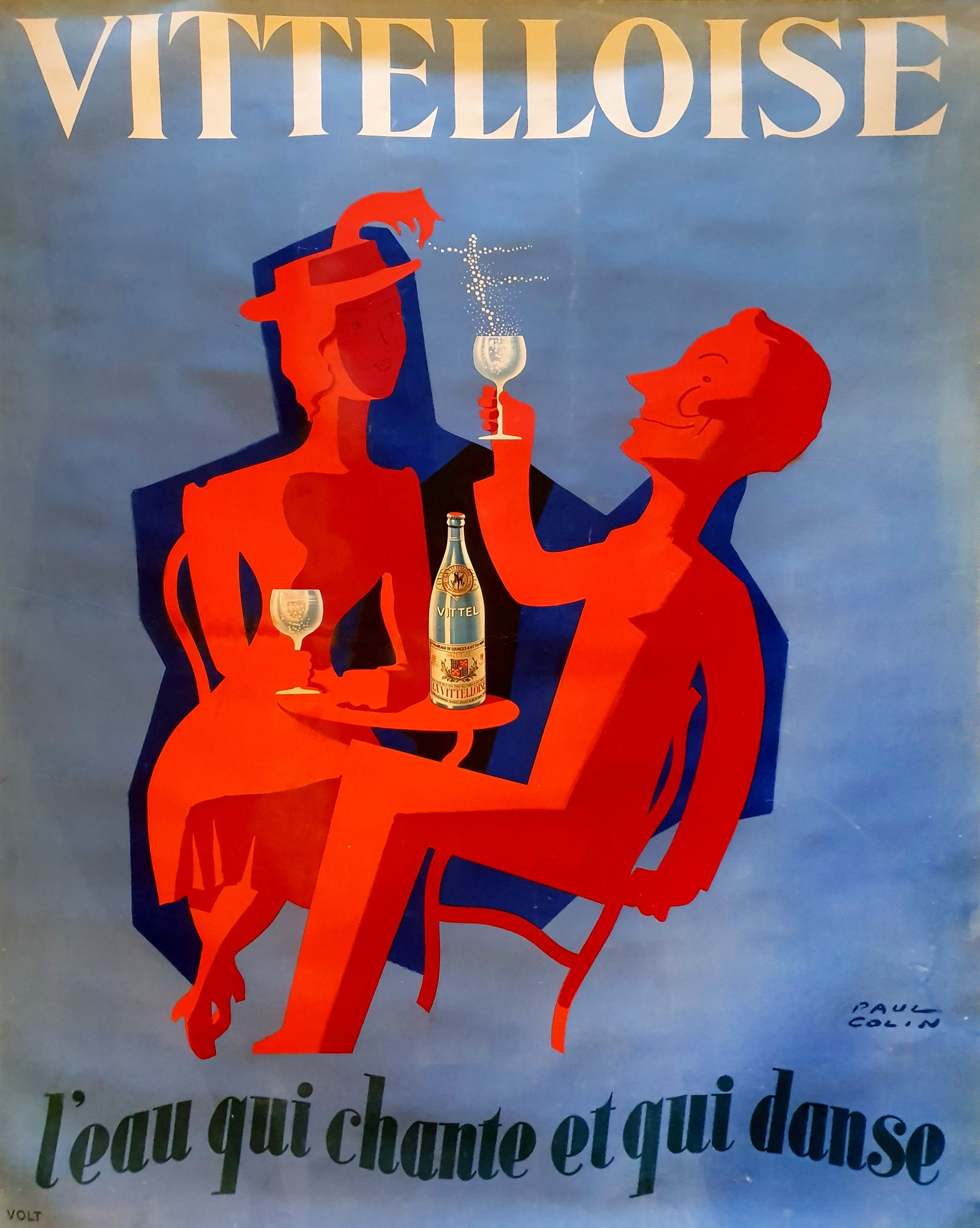This image is a poster featuring an abstract representation of a stadium event, prominently titled "Roland Garros 89" in dark blue, somewhat messy handwriting. The background transitions from a dull orange at the top to a brighter, more vivid orange at the bottom, suggesting the use of construction paper. At the center of the composition, there is a tilted, bright red rectangle, symbolizing the stadium itself. 

Surrounding this central rectangle are hundreds, if not thousands, of small blue, red, and white dots. These dots signify the crowd; closer inspection reveals details such as blue heads and white shirts that embody the spectators. Some dots are more defined, showing arms or suggesting female shapes. Inside the red rectangle, there are two distinct white spots—one elongated and another rectangular. These details collectively create a vibrant and dynamic depiction of people gathered in a stadium-like setting, possibly celebrating or commemorating an event at Roland Garros in 1989.